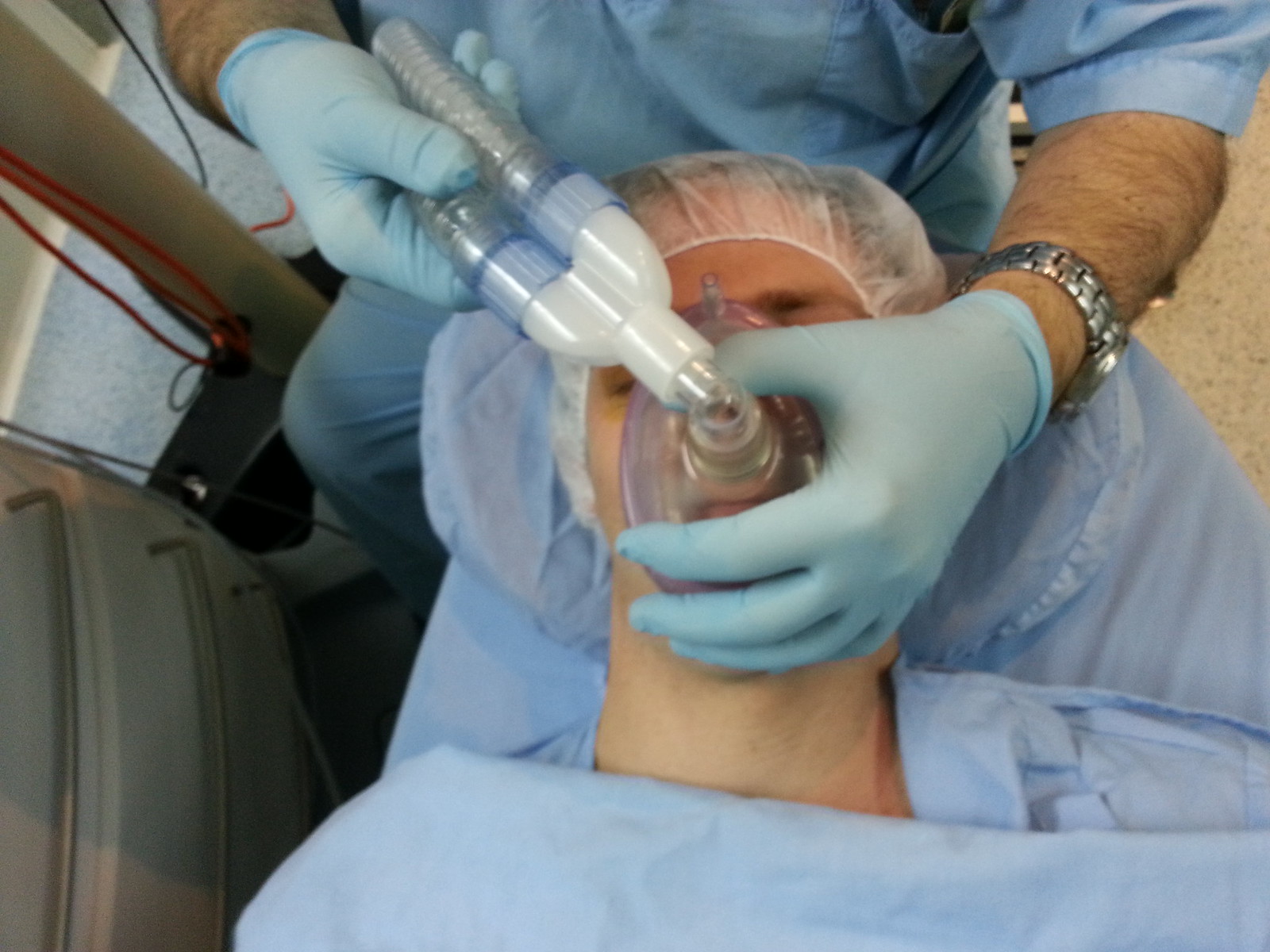The photograph captures a detailed scene in an operating room or medical setting. A woman lies on a blue sheet, wearing blue scrubs and a blue blanket with a hairnet covering her hair. Positioned from above, the image shows a man in matching blue scrubs and blue gloves, with a silver wristwatch on his left arm, holding a breathing apparatus over the woman's face. This apparatus is white with blue connections attaching it to a clear hose, likely for administering anesthesia or oxygen. The man is either standing or seated beside her, carefully applying the mask designed to help the woman breathe or sedate her. To the left of the scene, indistinct gray medical equipment, possibly a shelf and a standing device with a black base, partially enters the frame, likely supporting the medical procedure.